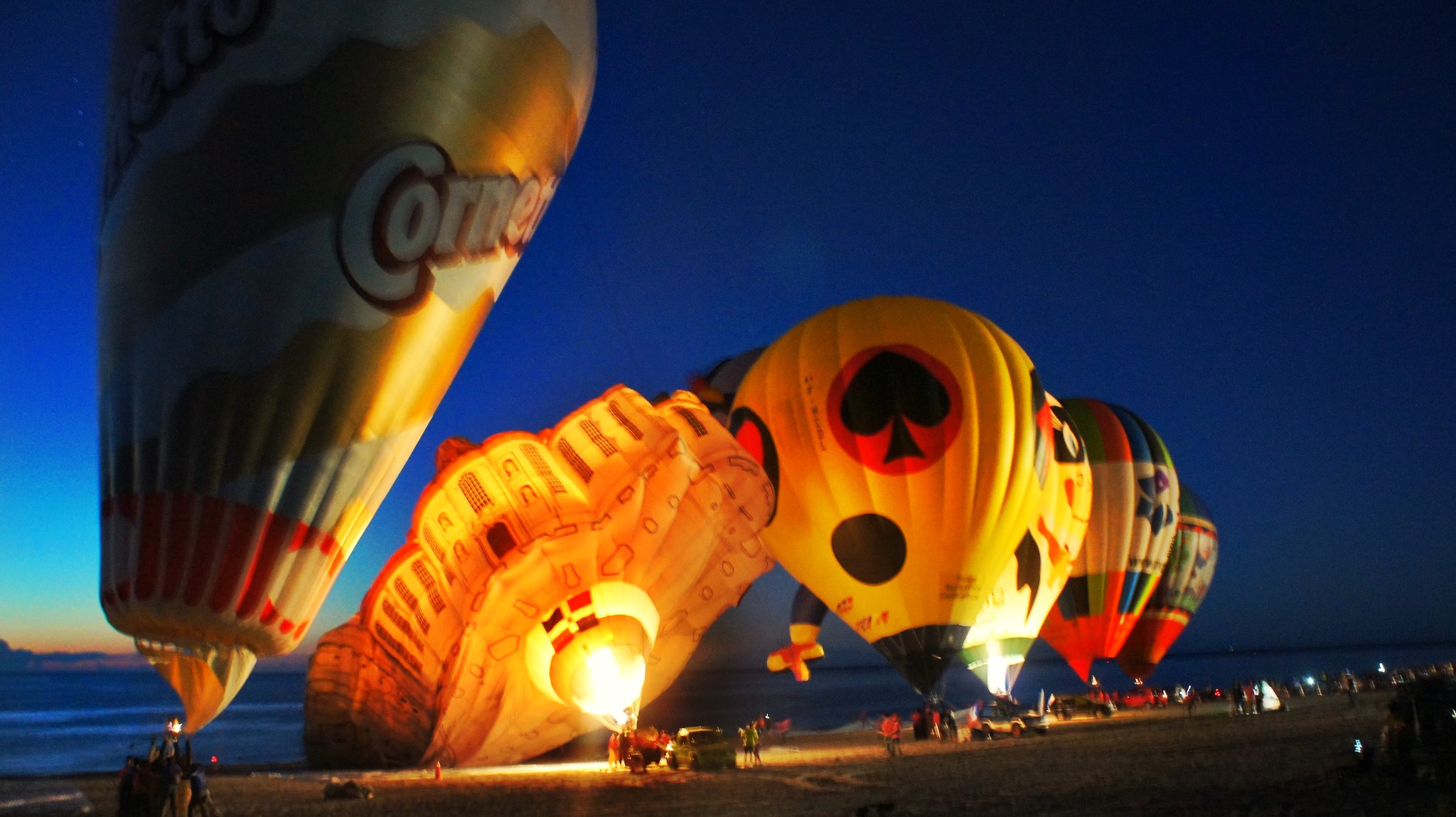The image depicts a vibrant scene of a beach at dusk, transitioning from the dark sapphire blue of the night sky on the right to a lighter aqua blue and orange on the horizon to the left. This tranquil skyscape meets a body of deep blue water in the backdrop. The foreground is lively, with a sandy beach bustling with people, cars, and tents. The main focus is on six large hot air balloons lined up in a row, their colorful designs and shapes captivating the onlookers. Starting from the left, the first balloon is gold and has the name "Cornet" on it, resembling an ice cream cone. The second balloon features a cityscape or carousel-like structure with a flame and a country flag beneath it. The third balloon has a cream yellow dome decorated with a black circle and a black heart encircled by red. Additional balloons display hues of blue, cream, and red, creating a striking visual against the serene evening beach scene.